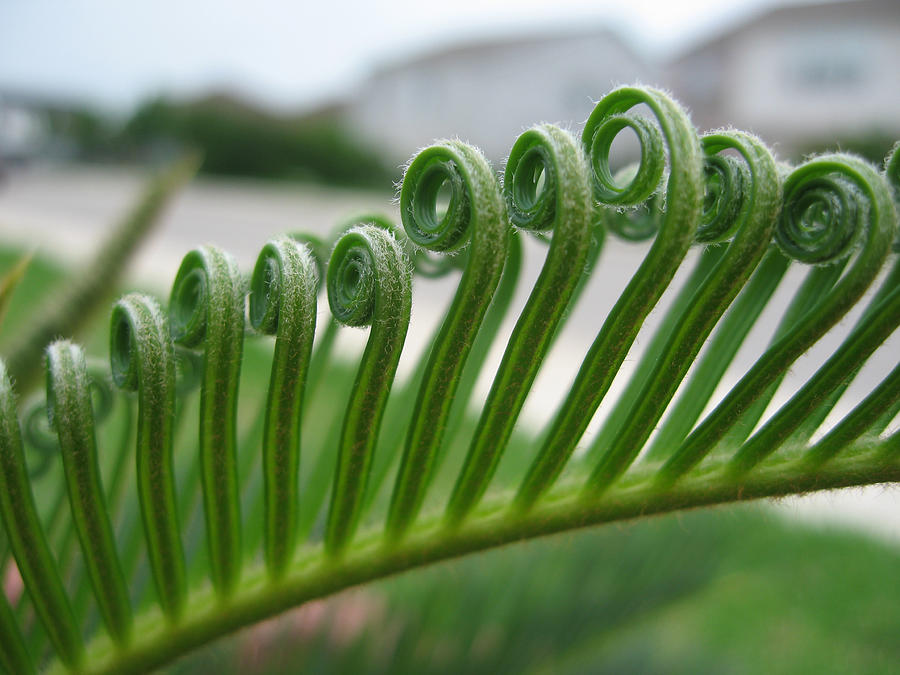This macro photograph exquisitely showcases a partial frond of a fern plant, emphasizing its fascinating structure and texture. Each long, thin leaf on the fern sports a distinctive, tightly wound spiral at its end, resembling delicate springs. The leaves, light green with a prominent dark green stripe running along their middle, are adorned with numerous small white hairs that follow the contours of the curls, adding a furry appearance to the plant. The thick stem of the fern, less prominent but still noticeable, supports over ten of these intricately curled leaves, arranged in rows with some partially obscured behind others. The background, intentionally blurred, hints at a neighborhood setting with the vague outlines of houses and a road, ensuring that the viewer's attention remains on the unique and captivating details of the fern's spiraled leaves.